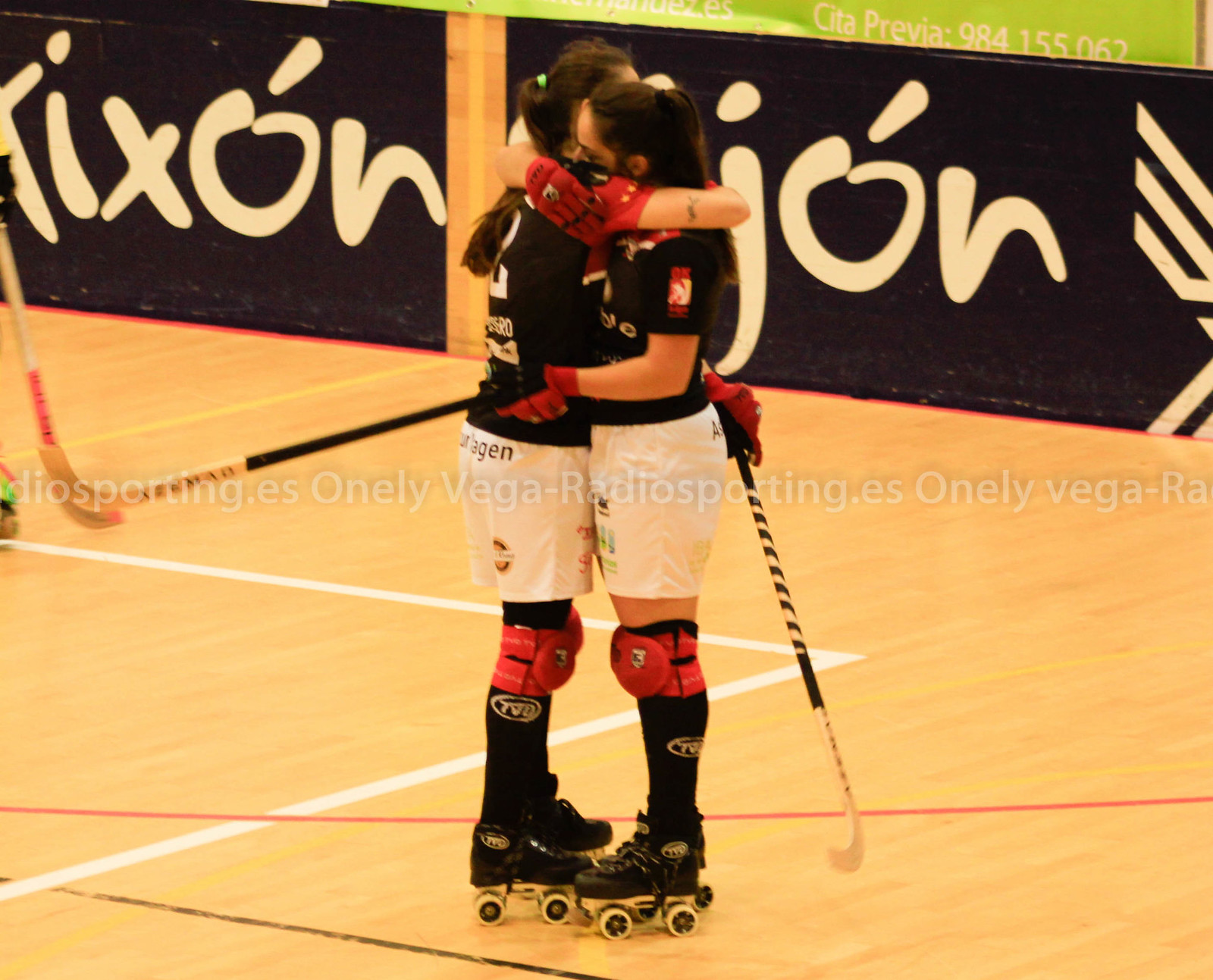This photograph captures an emotional moment between two female athletes, dressed identically in black jerseys with white numbers and red logos, and white shorts. They are equipped with red knee pads, high black socks, and traditional four-wheeled roller skates. Both women hold curved sticks, reminiscent of hockey sticks, suggesting they're engaged in a roller hockey game. The scene unfolds on a wooden sports court with visible white and red lines marking the playing area. In the background, there's a fence adorned with a partially visible white text that reads "I-X-O-N" and possibly "J-O-N," hinting at potential sponsors. The image is overlaid with a watermark that says "OneLeigh Vega R Radio Sporting dot ES," ensuring its originality and preventing unauthorized use.